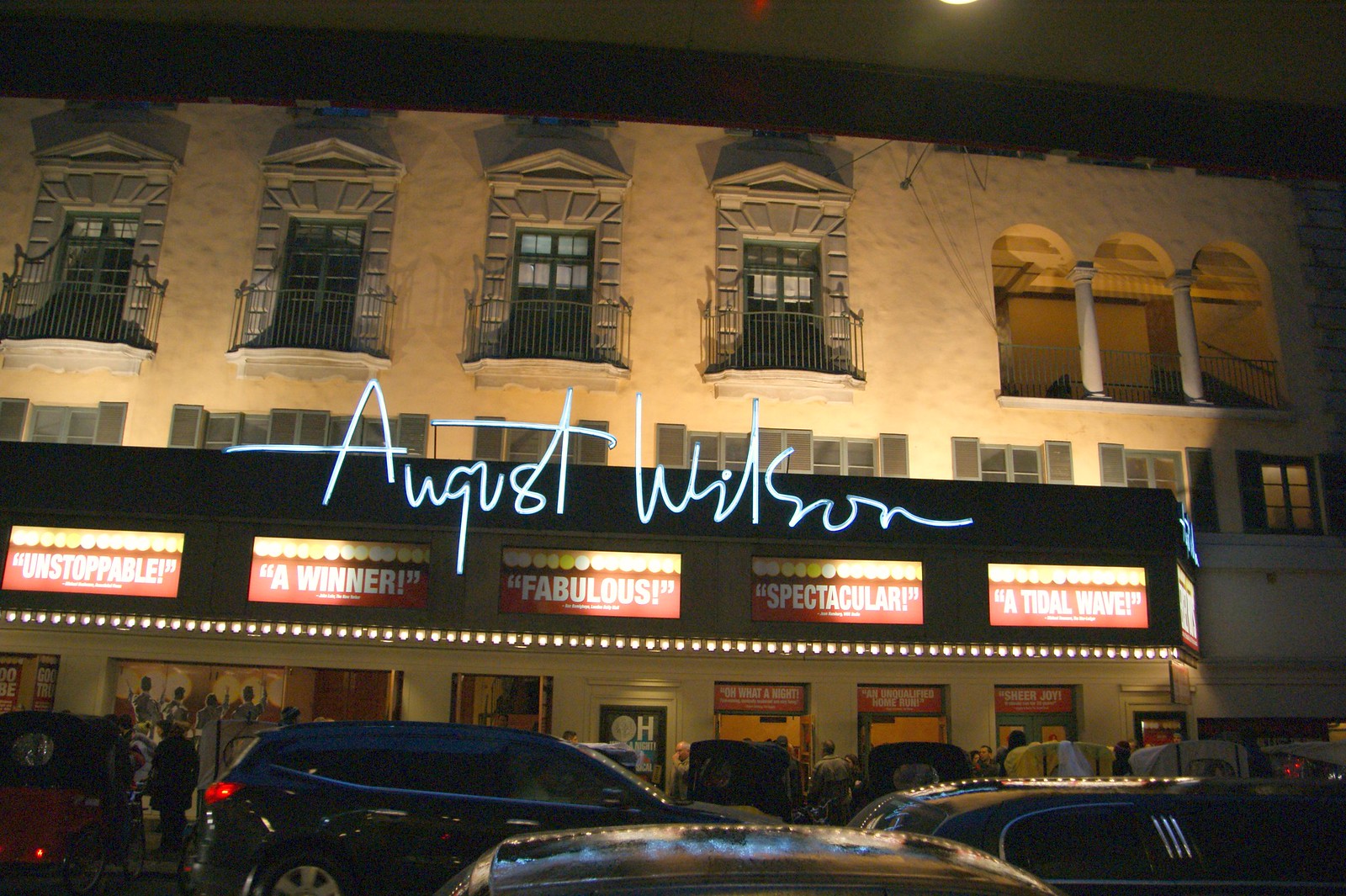The photograph, taken outdoors at night, captures an ornately designed, older-style building that resembles a grand old theater. The image is shot from across the street, evident by the two rows of cars and rickshaws visible in the foreground. The building's façade is lit up with bright lights, illuminating its intricate details and creating a striking visual against the dark sky. The architecture features four balcony window doors spanning from left to right and an open-air area with a balcony-like feel, although it is covered and situated within the building.

Prominently displayed in neon, white-ish cursive writing across the building’s front middle is the name "August Wilson," almost as if it were a signature written in lights. Below this signature, theatrical-style rectangular signs with a red background each feature dramatic descriptors outlined with round theatrical lights, reminiscent of those found around a dressing table mirror. The signs read: "Unstoppable," "A Winner," "Fabulous," "Spectacular," and "A Tidal Wave." 

Beneath these signs are ticket windows with people milling around, lining up, and moving in and out of the entrance. The street in front of the building appears to be a one-way street with diagonal parking, adding to the distinct foreground elements that include various pedestrians and rickshaws ready to offer rides.